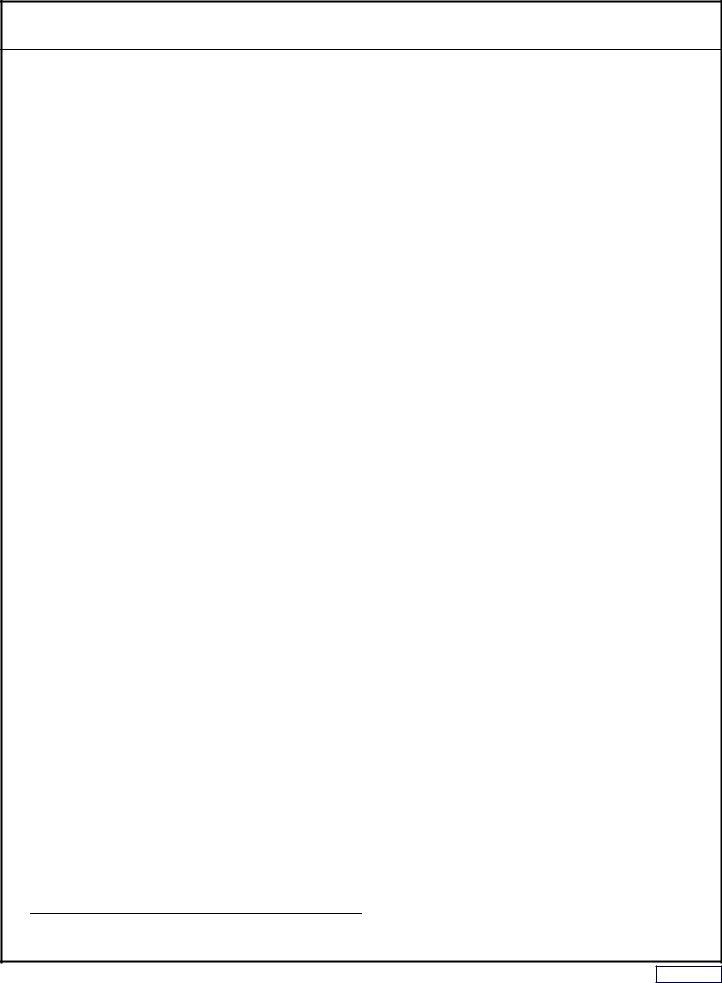Error Image Description:
The image currently displayed is not loaded properly, showcasing a black border surrounding a blank white center with a small black line within it. This appears to be an error, resulting in an unviewable or blank image.

Additional Context:
While describing the image, I was reminded of an exciting soccer match I watched recently. It was a Round of 16 clash between Portugal and Slovenia that extended into extra time. Despite a stalemate and vigorous gameplay, the score remained 0-0 by the end of extra time. Portugal ultimately triumphed in the penalty shootout, winning 3-0. This outcome was remarkable as the Portuguese goalkeeper managed the rare feat of saving three consecutive penalties that were on target. I was cheering for Portugal, and their victory in such a dramatic manner was both satisfying and extraordinary.